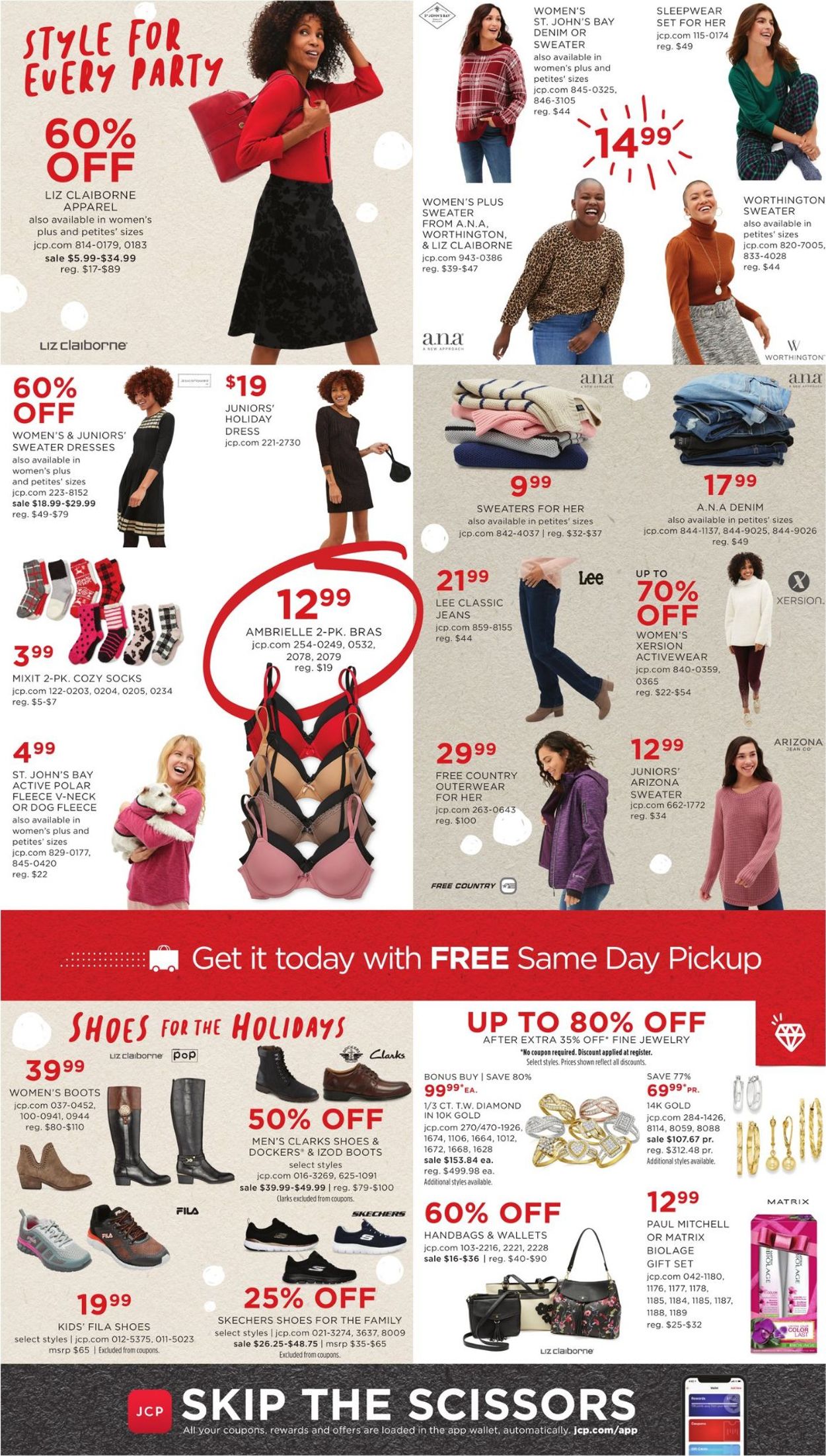This is an advertisement for a JCPenney clothing store, presented in an elongated vertical format with several distinct segments. 

At the very bottom of the ad, a red box prominently displays the text "JCP, skip the scissors," accompanied by an image of a phone, encouraging customers to clip coupons digitally onto their phones.

Above this, the advertisement is divided into six panels showcasing different products and offers:

1. **Top Left Panel:** A stylish woman is featured, dressed in a skirt and sweater combination, accessorized with a red purse.
2. **Top Right Panel:** Various clothing items are advertised at a reduced price of $14.99.
3. **Middle Left Panel:** A diverse assortment of children's clothing, socks, and bras is displayed, with the bras specifically highlighted by a red circle around the price of $12.99.
4. **Middle Right Panel:** There are sales promotions on women's pants and sweaters.
5. **Bottom Left Panel:** This section is dedicated to various shoes and boots, all of which are on sale.
6. **Bottom Right Panel:** An assortment of jewelry, purses, and hair care items is shown, all available at discounted prices.

Between the middle and bottom panels, a bold red stripe communicates, "Get it today with free same-day pickup," emphasizing the store's convenience and prompt service. This detailed layout showcases JCPenney's broad range of products and attractive sales, encouraging shoppers to take advantage of the digital coupon option for added savings and convenience.